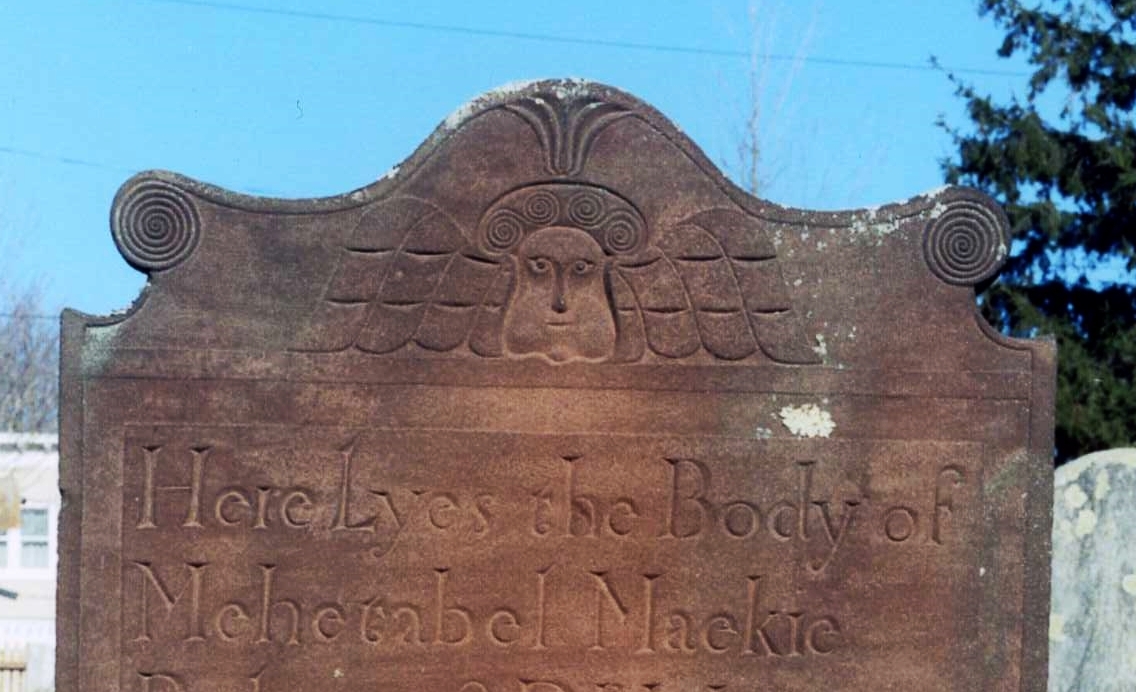This image features an aged, intricately carved headstone, prominently displayed in the center of the photograph. The headstone is a brownish or rust color, shaped with elegant curves and adorned with an elaborate design at the top, featuring a stylized face with angel wings, accompanied by swirling patterns. The inscription, hand-carved in the stone, reads "Here lies the body of Mahetna Bell Mackey," with "lies" notably spelled with a "Y." The photograph, taken during the daytime, captures a clear blue sky in the background, and to the right, a tall pine tree. A silver and white headstone is partially visible in the bottom right corner, while to the left, a white building with visible windows and hints of another tree can be seen. Additionally, power lines traverse the sky, adding to the scene's historical and somewhat somber ambiance.